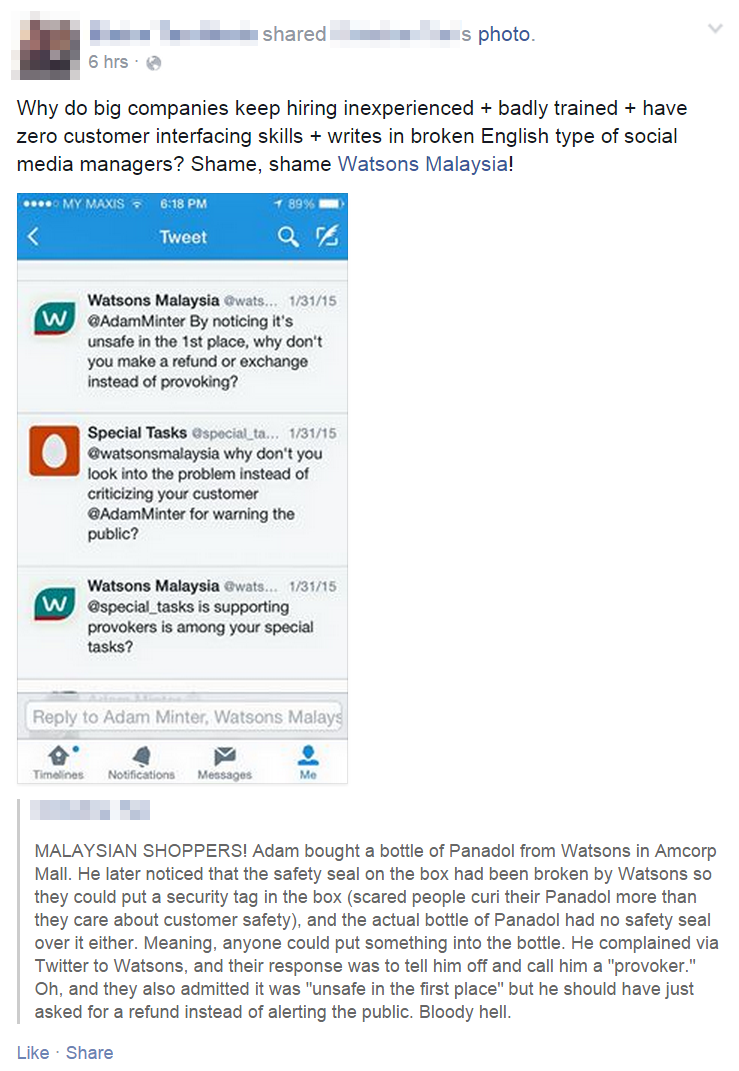**Caption:**

A blurred image reveals a series of tweets, with the usernames and profile photos obscured for anonymity. The first tweet criticizes Watsons Malaysia, questioning why large companies hire social media managers who lack experience, proper training, customer service skills, and proficiency in English. The tweet ends with a call-out: "Shame, Watsons Malaysia."

A screenshot of the tweeted conversation follows. It reads:

1. Watsons Malaysia @WATS 131.15 to @AdamMinter: "By noticing it's unsafe in the first place, why don’t you make a refund or exchange instead of provoking?"
2. Special Tasks @SpecialTasks 131.15 to Watsons Malaysia: "Why don't you look into the problem instead of criticizing your customer @AdamMinter for warning the public?"
3. Special Tasks again: "Is supporting provokers among your special tasks?"

Below the tweet series, additional text narrates the incident:
"Malaysian shopper Adam bought a bottle of Panadol from Watsons at Amcorp Mall. He later discovered that the safety seal on the box had been broken by Watsons to insert a security tag, raising concerns about customer safety over product securitization."